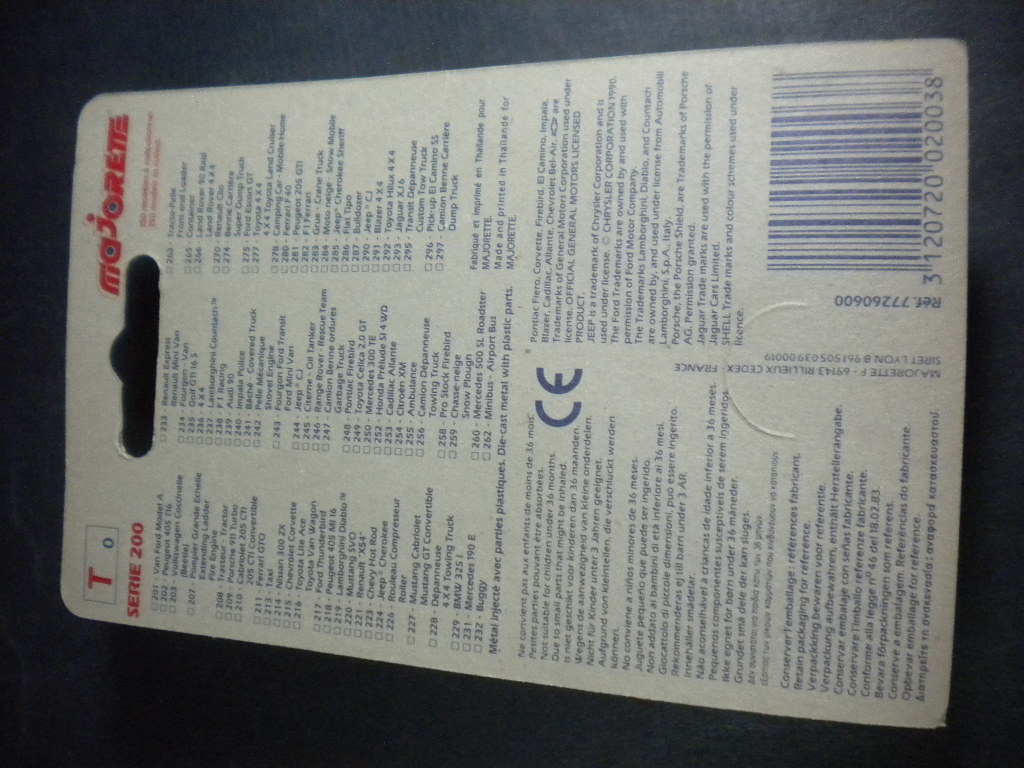This image features the back panel of a retail store toy package laid sideways on a black surface that exhibits subtle variations in lighting. The panel, primarily made of standard cardboard gray, is densely covered with blue text running vertically. In the top left (when oriented correctly), a prominent red "Majorette" or "Marjorette" branding is visible. The right side of the photo (top when oriented correctly) showcases a rectangular box containing "T Series 200." Below this, several rows list car names along with associated numbers. The lower section of the panel contains multilingual text, including phrases like "metal, inject, AVEC, parties, plastic, die cast metal with plastic parts." The middle of the panel has a CE mark with a circular design, and at the top right corner (bottom when oriented correctly), there's a UPC code. An oval cutout is present in the center, designed for hanging the package on a store peg.